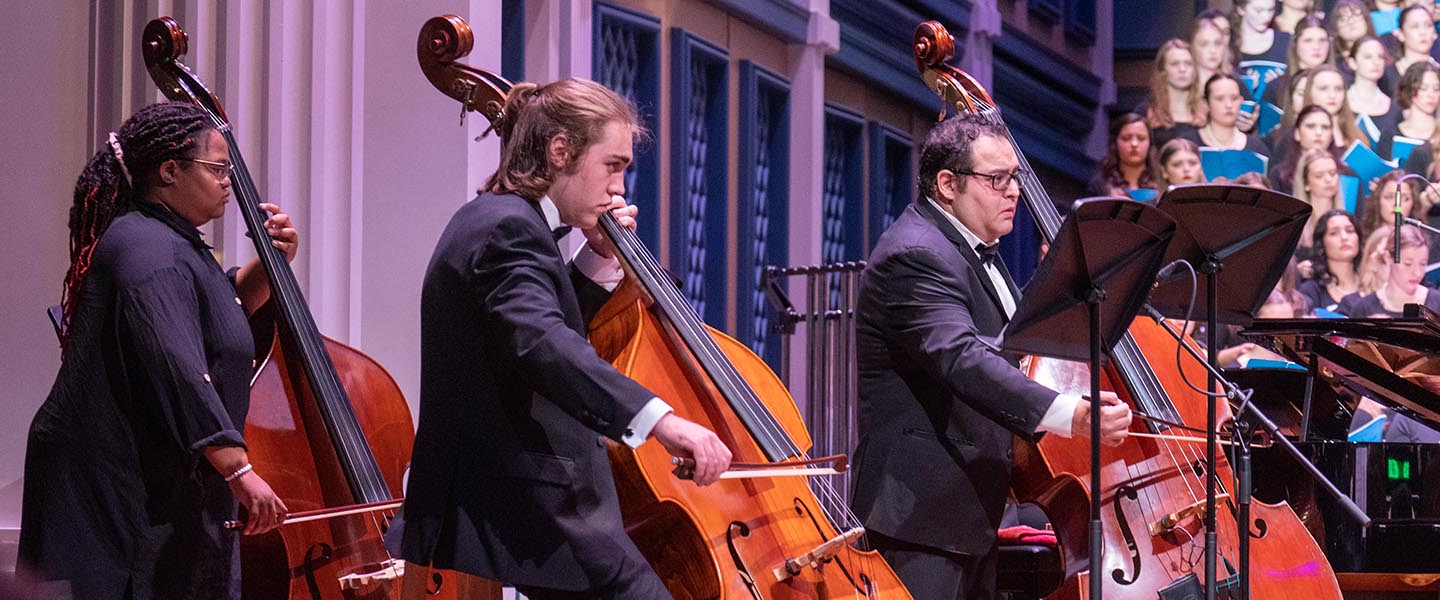In this detailed image of a musical performance, we observe a choir and a small orchestra in a very refined venue. On the right side of the image is a choir that consists entirely of women, all holding blue music books. They are arranged on risers and their faces are visible, focused on their performance. 

To the left of the choir, standing in a line, are three classical musicians. Each is playing a cello, indicated by the large, brown instruments that resemble oversized violins resting on the ground. All three musicians are dressed formally; two men and one woman, with the men donning black tuxedos and the woman wearing a black dress. 

The young male musician in the center stands out with his youthful appearance, long hair tied back into a small ponytail, and he appears to be leaning slightly as he plays. The man on the right, who is serious in demeanor, sports glasses and short black hair. To the left, the female cellist has long black hair, and all musicians hold their bows poised over the strings of their instrument.

In the background, the elegant music hall can be seen with large windows that form the backdrop of this performance. The scene is set on a stage, and a grand piano is partially visible to the right of the choir. The overall atmosphere exudes a sense of classic sophistication and the commitment of the performers to their craft.